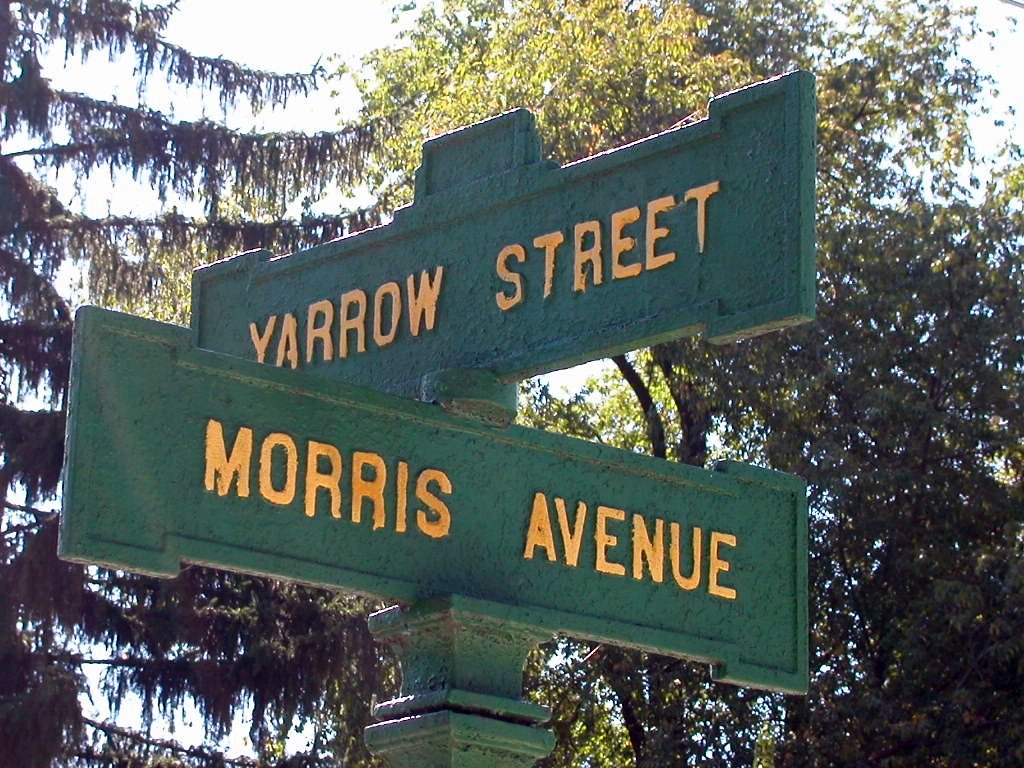This close-up image captures an ornately designed traffic sign situated on a decorative pillar. The hunter green sign points in two directions: straight ahead and back towards Morris Avenue, with Yarrow Street indicated perpendicularly. The sign's intricate design features raised and recessed edges, adding a touch of elegance. In the background, delicate conifer foliage and a lush, sunlit deciduous tree are visible, with patches of clear sky peeking through the leaves.